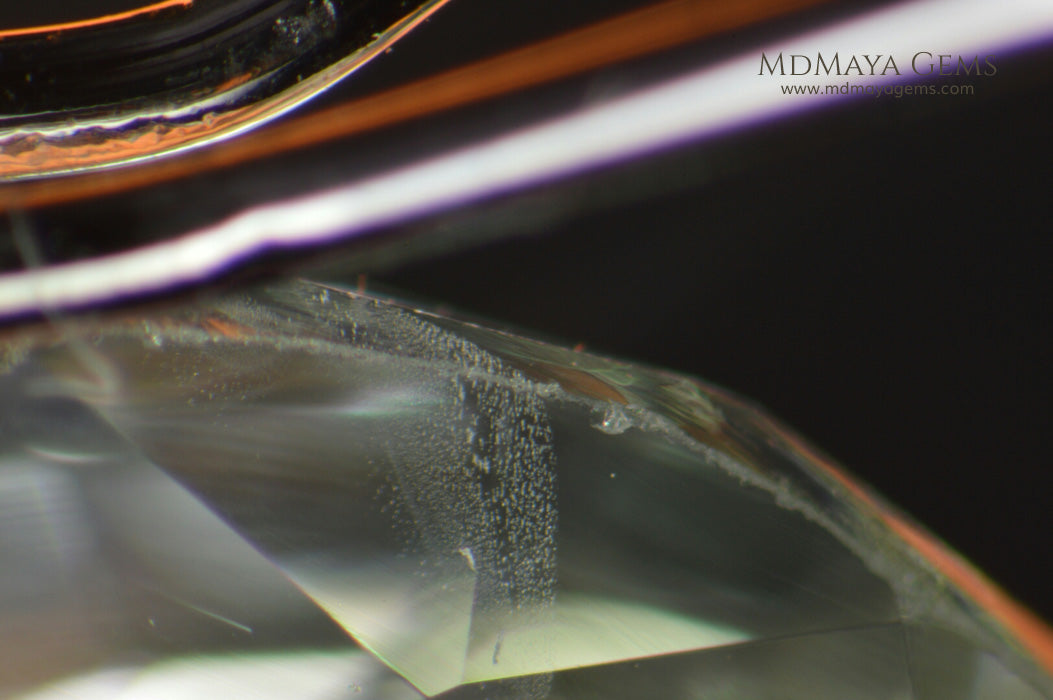The image is an extremely close-up photograph of a clear, faceted gem, possibly a diamond, revealing its intricate angles and flat surfaces. The bottom half of the picture is dominated by this glassy, diamond-like stone, showcasing its faceted structure with visible crevices and imperfections. The background is predominantly black, accentuating the gem's clarity. Horizontal lines—one white and one red—traverse the image from left to right, with an orangish light appearing above the white strip, hinting at the lighting or possibly another gem. In the top right corner, there is text that reads "MDMayaGems" alongside the URL "www.MDMayaGems.com." The combination of these elements suggests this is an advertisement or promotional image for a company specializing in high-quality gems, emphasizing the gem's detailed appearance as observed through a microscope.